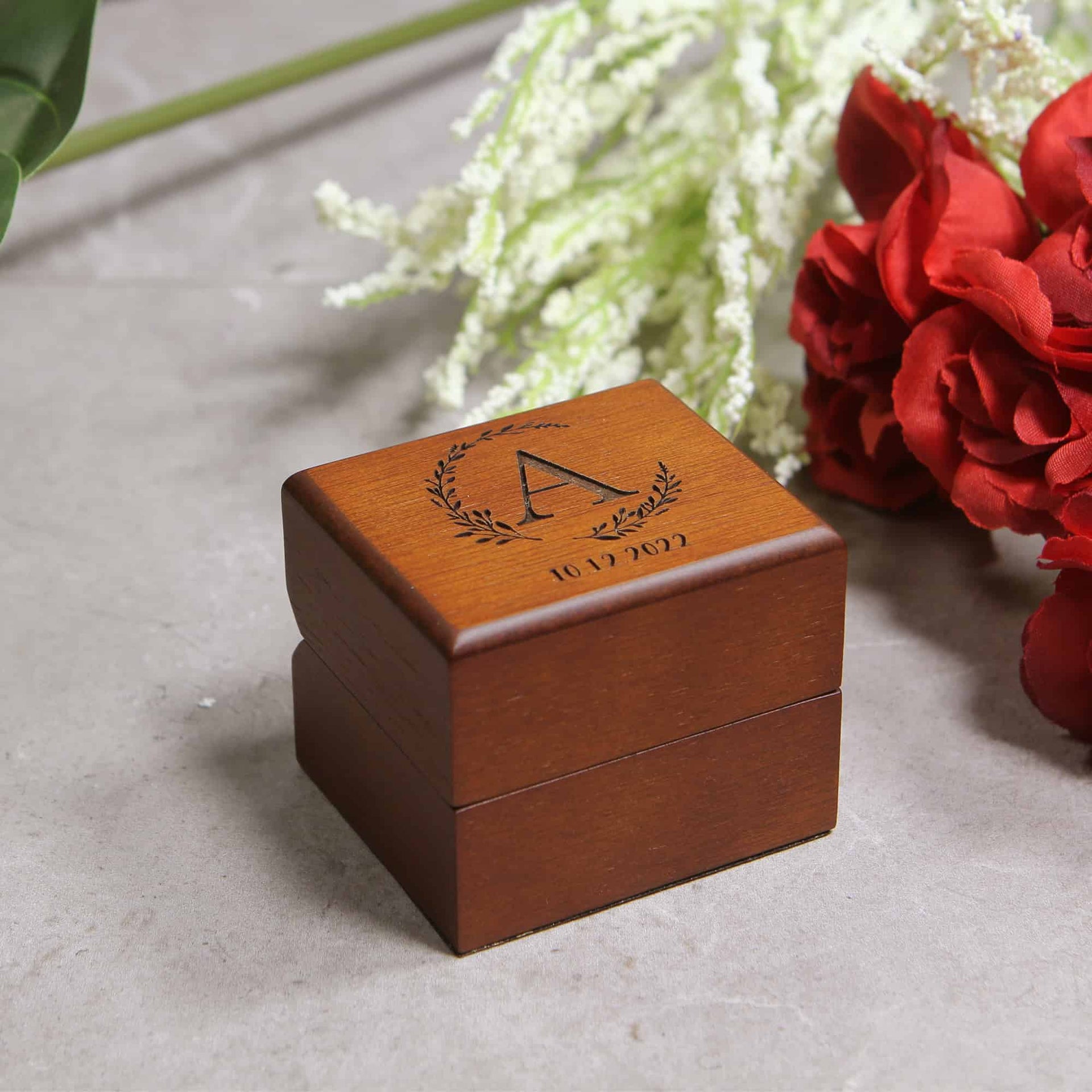The image depicts a small, mahogany-colored wooden box, centrally positioned on a gray table. The box has a smooth, reddish-tinted surface with beveled edges and features an engraved letter 'A' surrounded by olive leaves or similar foliage. Additionally, it is etched with the date 10-12-2022 in black. On the table around the box, there are various flowers: a bouquet of roses on the right, white flowers resting on top, and a greenish flower in the top left corner. This setting, likely part of an engagement or wedding scene, showcases the box which is presumably designed to hold a proposal or wedding ring.